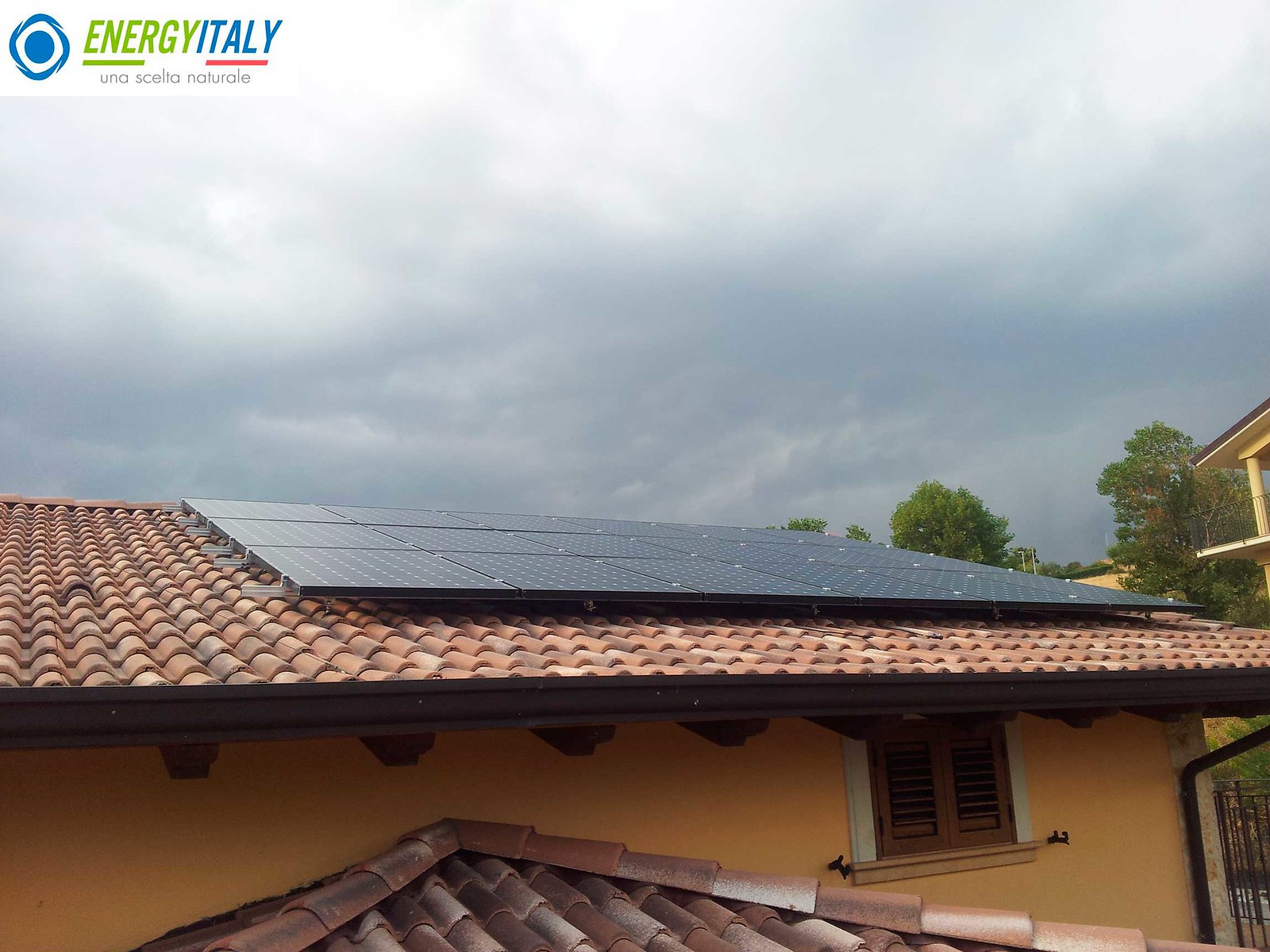The image depicts an Italian scene on a cloudy day with dark, threatening skies. Prominently featured in the upper left-hand corner is the text "Energy Italy" with the phrase "U.N.A. S.C.E.L.T.A. N.A.T.U.R.A.L.E" written below it. Dominating the lower half of the picture is an orange house with a terracotta roof. The roof is notable for its 18 black solar panels, laid out in a grid pattern, designed to harness solar energy. The unique roof design appears to be a wedge type and is accompanied by black gutters. Just below the roof, a window with shut blinds is nestled within a wooden frame. The house has a substantial overhang, creating an awning effect, and there's a glimpse of a secondary roof or porch area. Off to the right, the scene includes trees and the tops of other buildings, adding context to this residential setting. The overall atmosphere suggests an imminent rainstorm, emphasizing the dark and cloudy sky above.